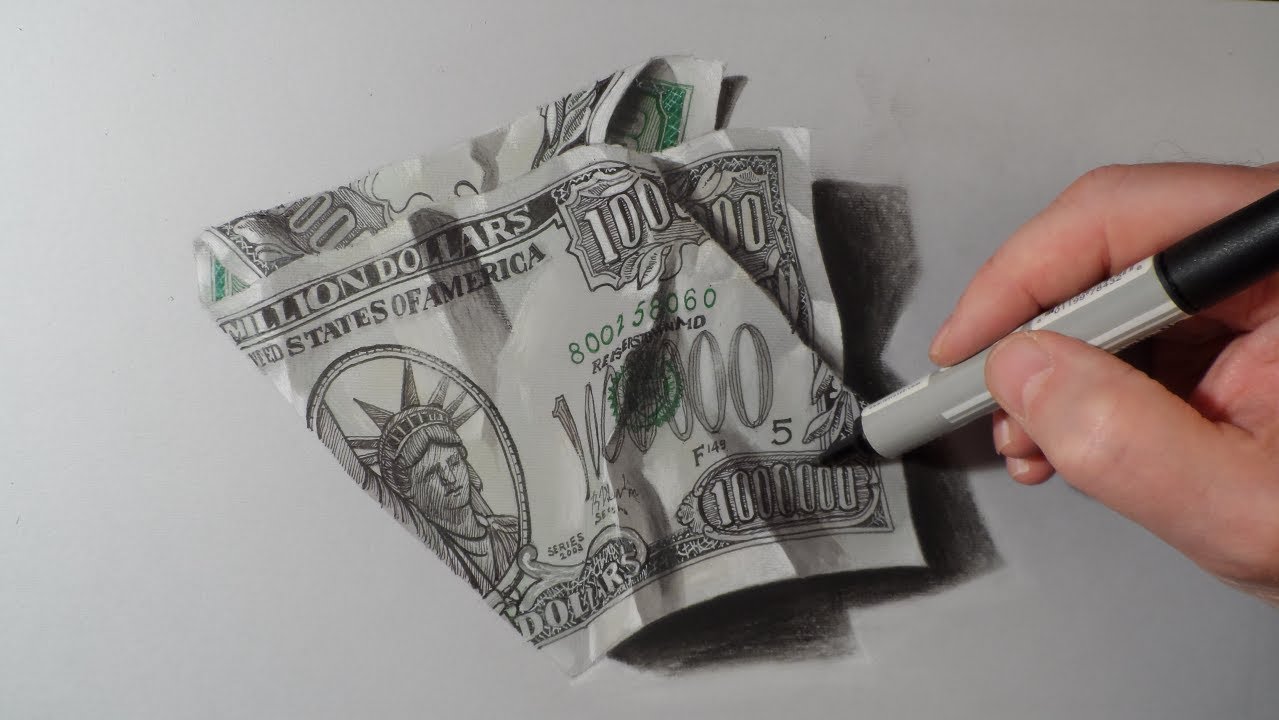In the photograph, a crumpled counterfeit $1,000,000 bill is prominently displayed on a grayish tabletop. In place of a presidential portrait, the center of the bill features the Statue of Liberty. The bill conspicuously showcases "$1,000,000" at the top, along with "United States of America," and a serial number, 800258060. A person's right hand, partially cut off from the frame, is seen holding a black Sharpie at the bottom right corner of the bill, poised to write or sketch. The detailed design of the bill, despite being counterfeit, gives it a realistic appearance.